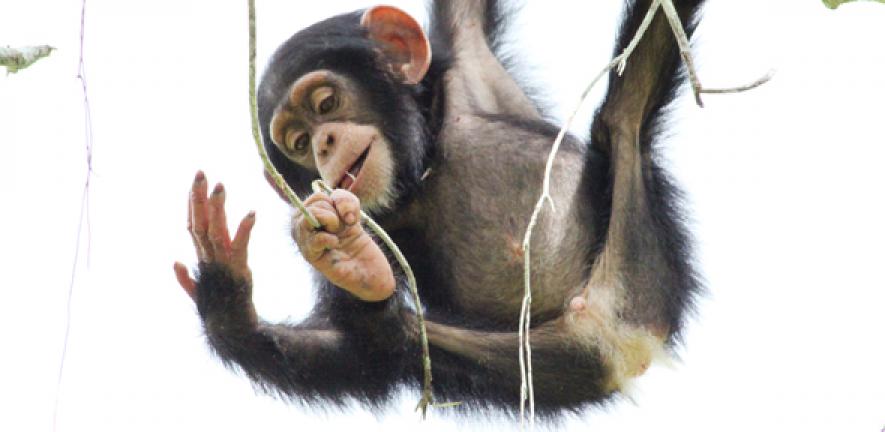This detailed photographic image, set against a completely white background, captures a baby chimpanzee with dark brown to black fur. The young male chimpanzee, appearing to be only a few days old, is hanging playfully from a green vine. The chimp's positioning features its head in the top left corner, gazing down towards the bottom left corner, while the rear points to the bottom right. Its legs are splayed, with the right foot clasping the vine firmly, and the left limbs partially visible. Notably, the chimpanzee has prominent light tan ears, and its open right hand is raised as if inspecting it. This delightful scene is devoid of any textual elements, highlighting the chimpanzee's playful and curious nature.